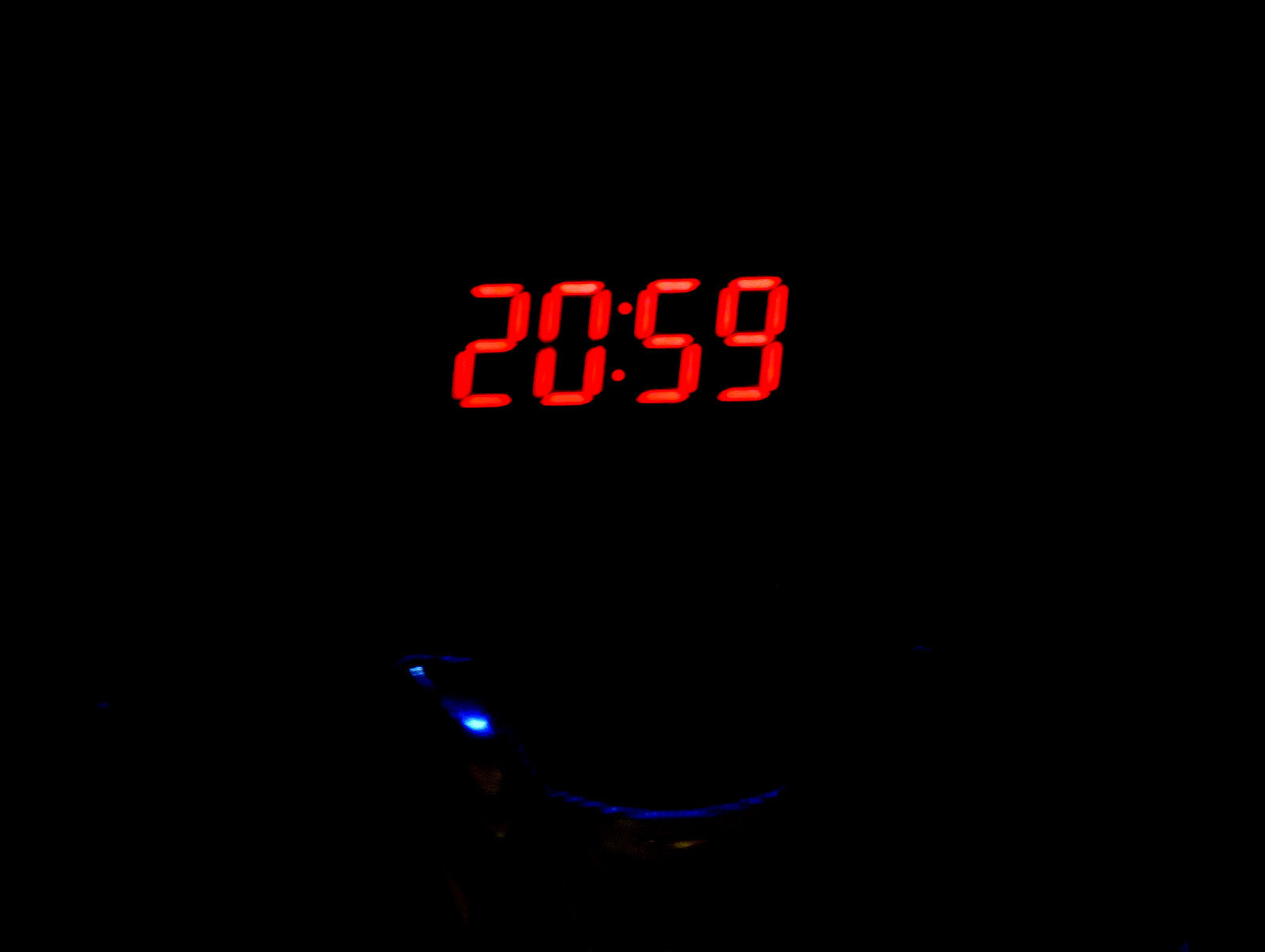The image is extremely dark, with an almost completely black background. At the center, the focal point is a slightly fuzzy, old-style digital clock display in red, showing the time 20:59. The numbers, which have a blocky design, exhibit a faint yellowish reflection. Below the clock, there's a light blue semi-circle reminiscent of an upside-down smiley face, accompanied by two bluish circles to the left. Additionally, a small, indistinct blue dot and an orange light are visible beneath this semi-circle.